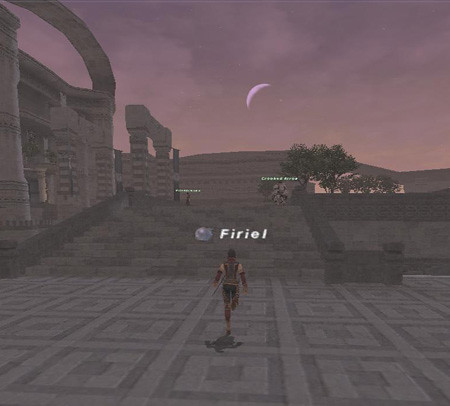In this computer-generated square image, a solitary figure is depicted in the lower center, captured mid-run with the back facing the viewer. The figure is clad in a white short-sleeved shirt adorned with a design or an accessory on top, paired with dark-colored shorts. The ground beneath them features gray square tiles set against a light purple backdrop. Directly in front of the runner is a set of wide stairs of a matching hue, ascending to another level. The architecture in the scene consists of stone or masonry buildings clustered to the left of the center, extending up to the upper left corner of the image. The sky above is enveloped in wispy, thin clouds, painted in shades of pink and gray, signaling a cloudy atmosphere. A crescent moon gently illuminates the scene from its position above a distant building, adding an otherworldly touch to the overall ambiance.